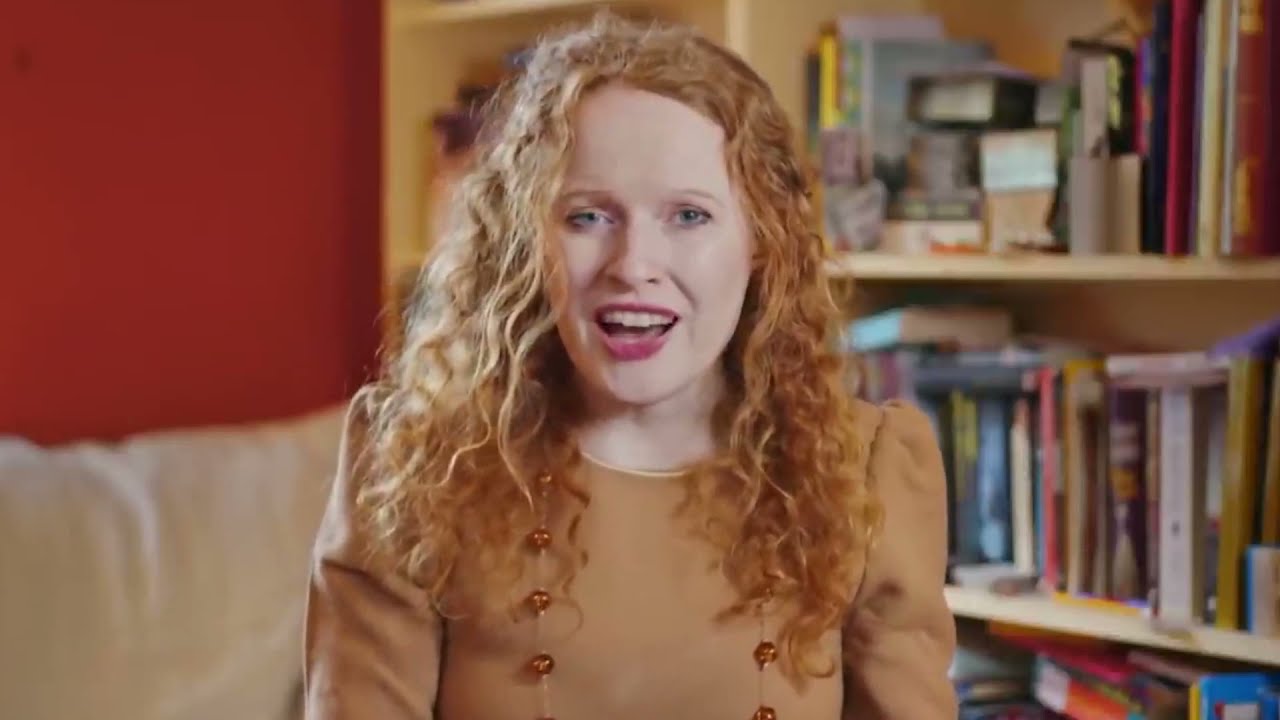In the photograph, a pale white woman with curly, strawberry blonde hair cascading just past her shoulders is captured mid-speech, her mouth partially open. She wears pink-red lipstick and light-colored, expressive blue eyes. Her attire is a tan, camel-brown long-sleeved outfit featuring a gold necklace adorned with amber-colored beads. The background reveals a room with a slightly out-of-focus mix of furnishings and decor. To her left, a reddish-orange wall provides a warm contrast, while to her right, a large, light tan bookshelf filled haphazardly with well-used books draws attention. The books, stacked both vertically and horizontally, hint at frequent use. A tan couch or chair is also visible in the background, enhancing the cozy, lived-in ambiance of the space.